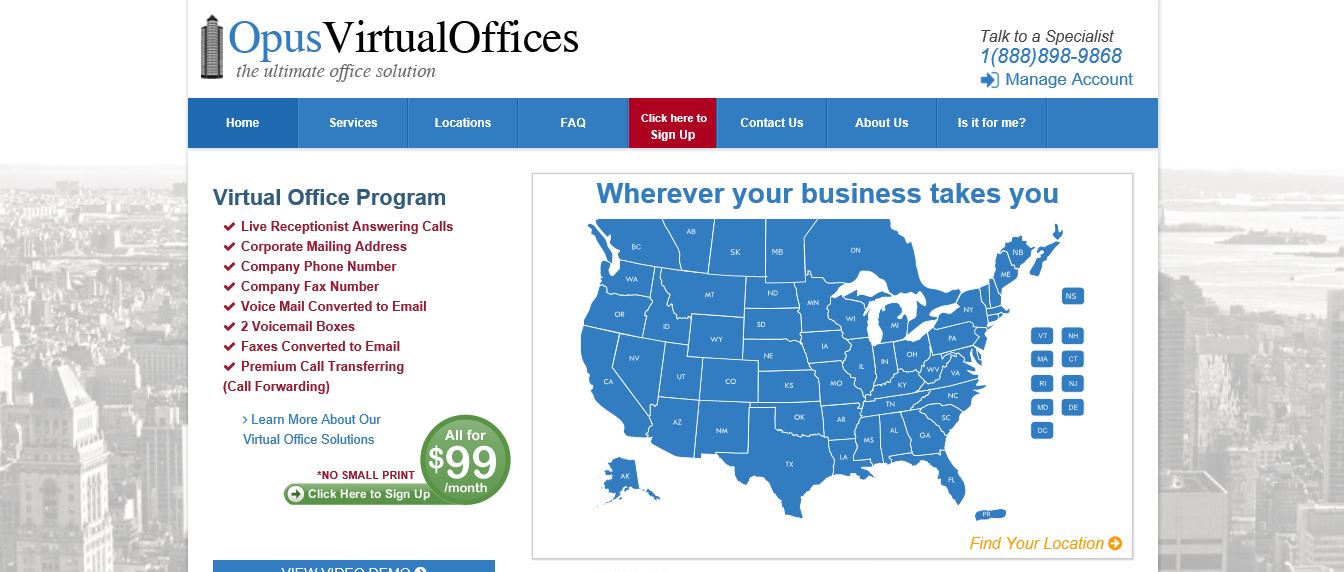The image features two prominent elements. The background is a grayscale aerial view of a city, showcasing towering buildings and a body of water. Overlaid prominently is a rectangular graphic occupying most of the page.

In the top left corner of this graphic, there's a picture of a tall building paired with the boldest text on the page, reading "Opus Virtual Offices." Directly below that, a subtitle states, "The Ultimate Office Solution." The top right corner of the graphic includes the text, "Talk to a Specialist," followed by a phone number, and then "Manage Account."

A blue border spans the width of the page beneath this, featuring multiple tabs. The first tab, highlighted in a darker blue, says "Home." The subsequent tabs read "Services," "Locations," and "FAQ." A red segment highlights "Click Here to Sign Up," and the blue background resumes with tabs labeled "Contact Us," "About Us," and "Is It for Me."

On the left-hand side, there's a column titled "Virtual Office Program" with checkmarks next to the following features: "Live Receptionist Answering Calls," "Corporate Mailing Address," "Company Phone Number," and additional details. This section highlights a price point, stating "All for $99."

To the right, there's an image of the United States with all states in blue and the Great Lakes in white. Above this map, the text reads, "Wherever Your Business Takes You." In the bottom corner, it says "Find Your Location."